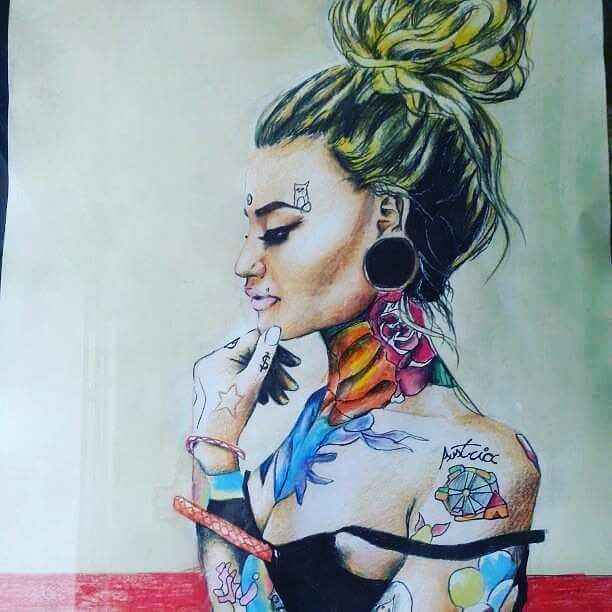This colored sketch portrays a woman with a vivid array of tattoos. She stands in a near-profile position, showcasing the intricate and vibrant designs inked across her body. Her neck is adorned with colorful tattoos, including flowers such as a rose in red and another in orange. She wears a black bra top, with one shoulder strap casually slipping off her shoulder, adding to the relaxed yet edgy vibe of the illustration.

Her hair is styled in a voluminous bun, predominantly black but accentuated with striking yellow highlights, reminiscent of blonde streaks. The woman's hand is elegantly posed with her chin resting on her knuckles, revealing more tattoos on her fingers and hand. Her facial features are notably striking, with very defined eyebrows and heavy eye makeup, characterized by a bold eyeliner on her upper lash line. Her lips are full and painted in a frosted white, adding to her dramatic and stylish appearance.